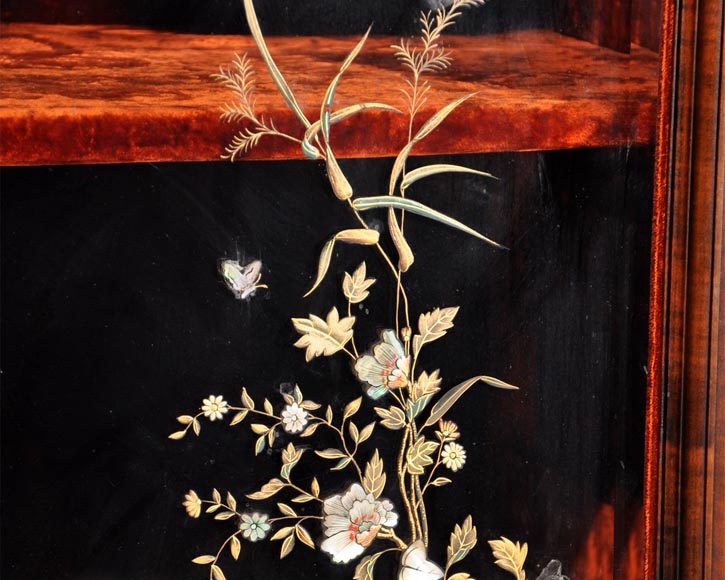The image features a detailed flower design that appears to be painted on glass. It's quite zoomed in, making it unclear what type of furniture the glass is part of, but there's a wooden edge on the right side, suggesting it might be a cabinet or a shelf. The top of the furniture is adorned with a red, possibly velvet material, adding an elegant touch.

The flower design consists predominantly of white flowers with touches of tan and gold, and possibly orange on the outside of the petals. These flowers feature red dots in their centers and green parts in the middle. Additional smaller flowers, in colors such as white, yellow, and green, with smooth or ridged leaves, accompany the main flowers. Another plant with long, grass-like leaves and a bud with wheat-like projections is also part of the composition. There is a butterfly depicted near the flowers, either about to alight or having just departed, adding a dynamic feel to the artwork. The background is entirely black, emphasizing the intricacy and colors of the flowers and plant elements.